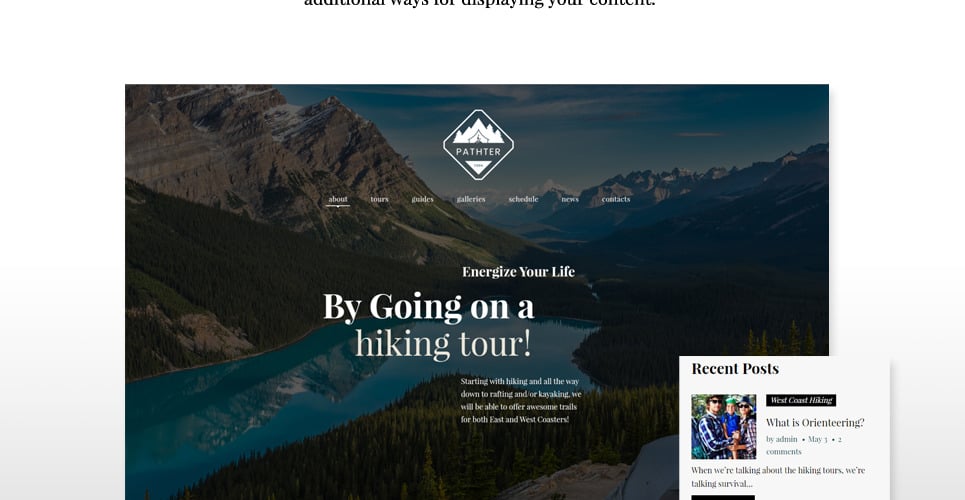**Descriptive Caption:**

This image captures a detailed screenshot of a nature-themed webpage. Dominating the page is a large, scenic image of a sprawling valley nestled between towering, green-covered mountains. The landscape features a mix of dense forests and rugged rock formations, all cloaked in a slightly dark filter that enhances the dramatic, serene beauty of the scene. A calm, blue lake mirrors the surrounding mountains, adding a tranquil element to the right side of the image. Among the trees on the right, there's a noticeable rock outcropping, possibly sheltering a tent, hinting at outdoor adventure.

The webpage headline reads "Energize your life by going on a hiking tour," which entices visitors with activities ranging from hiking to rafting and kayaking. A logo at the top of the page presents a minimalist design: a small tent beneath stylized white mountains, reinforcing the outdoor adventure theme. 

A navigation menu is prominently displayed, offering links to sections such as About, Tour Guides, Gallery, Schedule, News, and Contacts. In the lower right corner of the page, there’s a section labeled 'Recent Posts,' featuring links to articles like "West Coast Hiking" and "What is Orienteering?" by an admin, orienting readers towards hiking and survival topics.

Additionally, a smaller square image shows a family—a mother, father, and child—dressed in hiking gear, ready for an expedition, further emphasizing the family-friendly and adventurous spirit of the site.